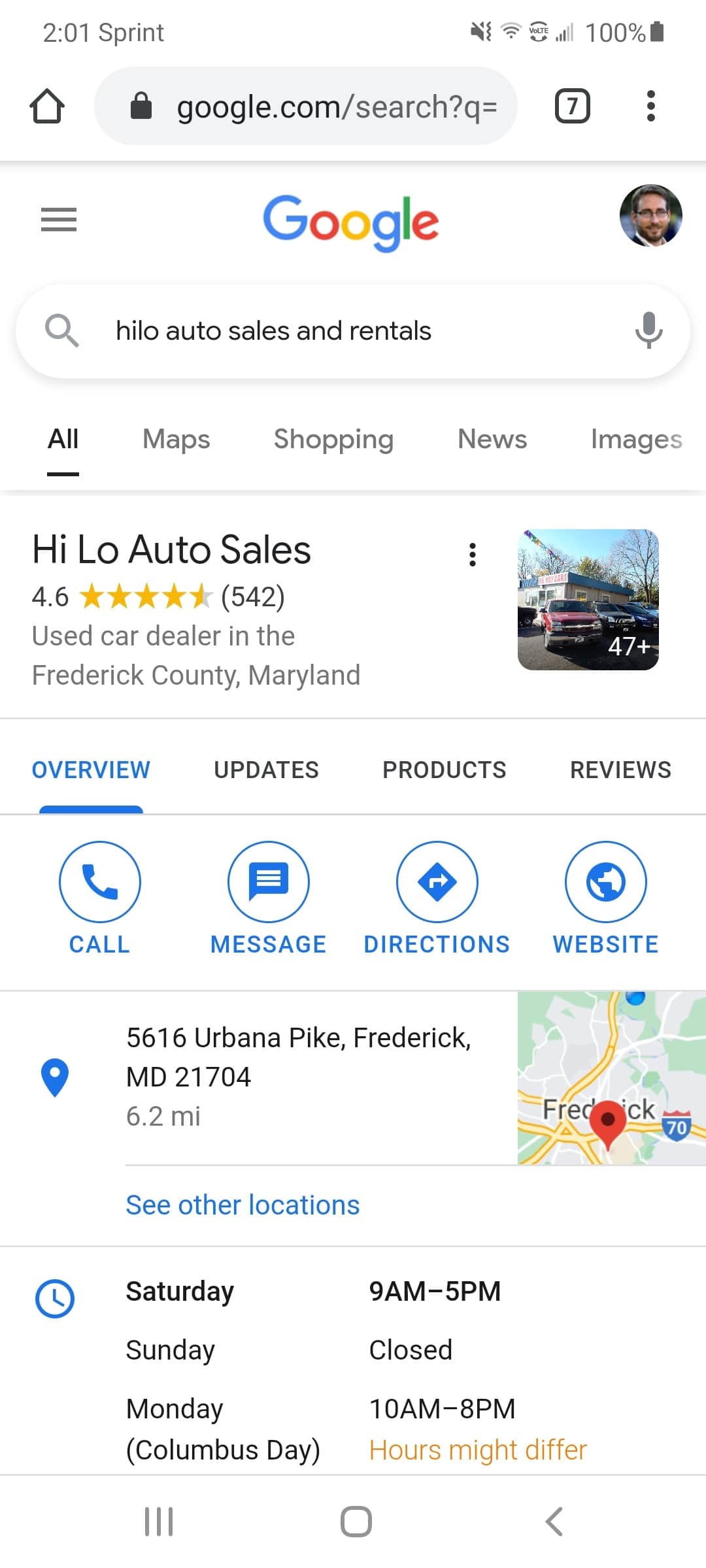This image is a detailed screenshot from a smartphone, captured in portrait orientation. At the top of the screenshot, there is a white notification bar separated by a thin gray line. In this bar, the current time is displayed as "201" in French. Additional icons indicate that the phone is on silent mode with vibration only, has full cell service, Wi-Fi connectivity, and a 100% fully-charged battery.

Below the notification bar is the Google search interface. The browser URL appears as "Google.com," and seven open tabs are indicated. There is a user's avatar on the right and the central Google logo featuring its characteristic colors: red, blue, yellow, and green. Directly below the logo, a search query for "Hilo auto sales and rentals" is entered, spelled "H-I-L-O."

The search results are displayed beneath the query, starting with an icon of a car next to the business name "HILO Auto Sales." The business is rated 4.6 stars. Further options to explore such as "Overview," "Updates," "Products," and "Reviews" are available, with "Overview" currently selected. The overview section presents the business's address and a pinpoint on the map, along with their operating hours.